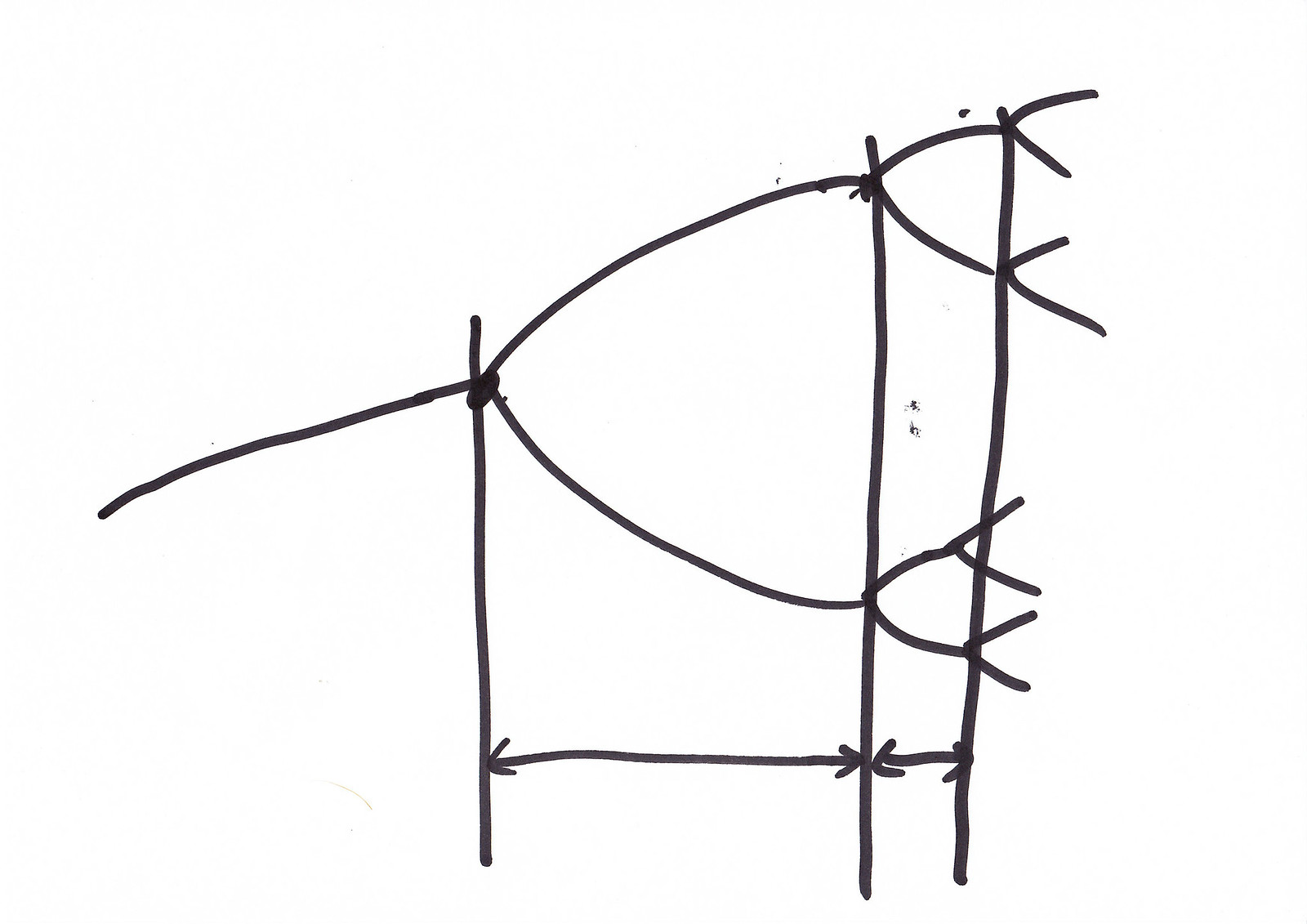This image seems to be a simple digital drawing, likely created using a computer application like Microsoft Paint. The picture features a stark white background with various black lines forming the entire composition. Three vertical lines dominate the scene, placed at specific intervals from left to right. 

Starting with the leftmost vertical line, which is approximately 2.5 inches tall, it sets the initial frame of reference. Moving about 2 inches to the right, another vertical line stands taller at around 3 inches. The last vertical line appears roughly half an inch to the right of the 3-inch line, and it is slightly taller than both previous vertical lines.

There are several diagonal lines creating a series of connected V shapes, adding complexity to the arrangement. The first diagonal line attaches to the top of the leftmost vertical line and extends to the second vertical line, forming the first V shape. From the top of this middle vertical line, another V shape extends to connect to the rightmost vertical line. A final, smaller V shape breaks off from this to continue further right.

Mirroring this series of V shapes, a similar structure exists at the bottom of the vertical lines, maintaining symmetry in the layout. Additionally, there is a horizontal line running along the bottom between the left and middle vertical lines, featuring arrows at both ends. Another horizontal line with arrows spans the gap between the middle and rightmost vertical lines, ensuring the design feels balanced.

This black-and-white drawing, with its intentional use of lines and spacing, appears well-structured despite its simplicity.